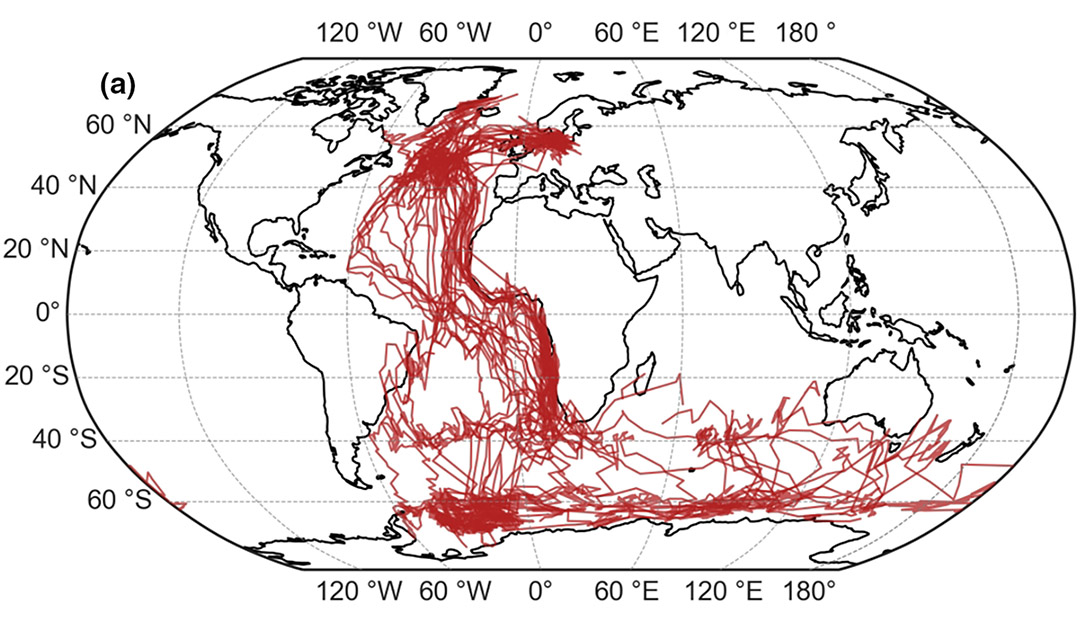This detailed drawing illustrates a world map rendered predominantly with black lines on a white background, enhancing its clarity and simplicity. The map, which is designed in an oval shape with flat borders on the top and bottom, features clearly marked continents and extensive latitude and longitude lines. These coordinates are prominently displayed around the oval, including degrees such as 120°W, 60°W, 0°, 60°E, and 120°E.

Within the map, vibrant red lines meander across the oceans in a seemingly haphazard manner, covering regions such as the waters between America and Africa, as well as those between Antarctica and Africa and Australia. These red lines possibly represent travel routes or shipping lanes, emphasizing their passage exclusively over water, without crossing terrestrial boundaries. For educational purposes, the precision of these details suggests a potential application in geography or navigation studies, highlighting the interconnectedness of global maritime routes.